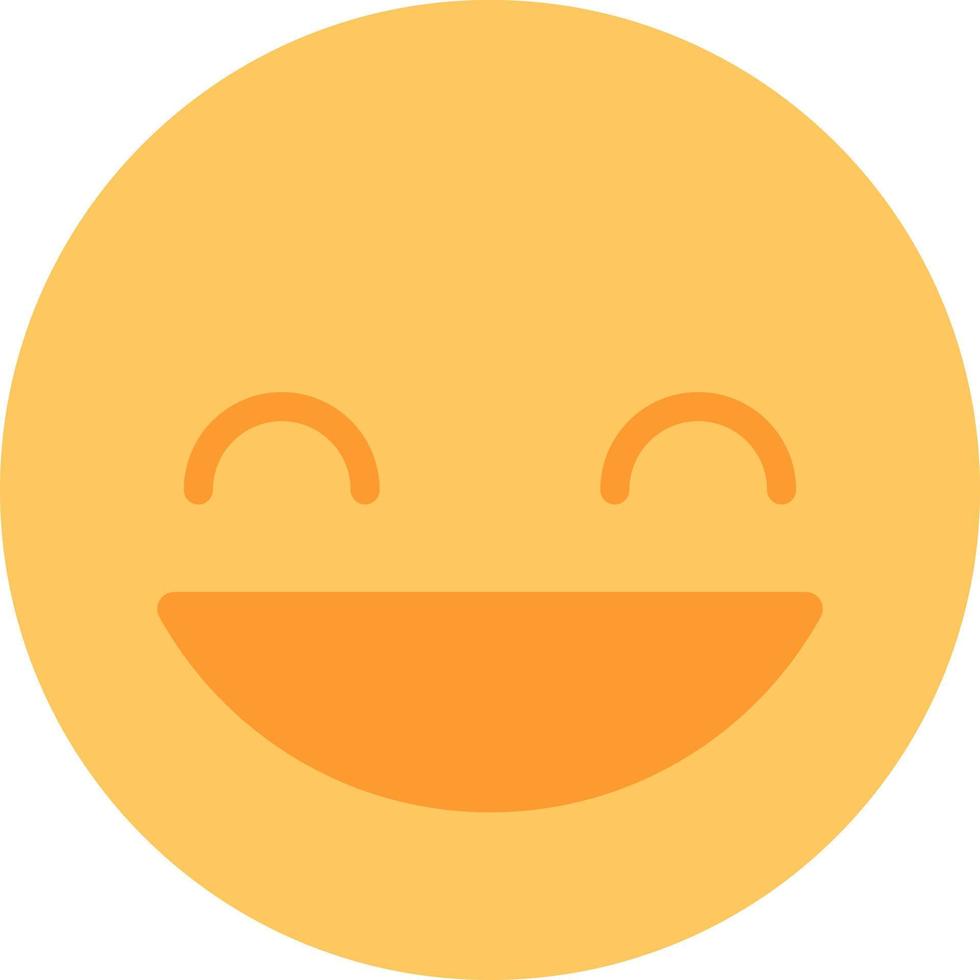This image depicts a classic, universally recognizable smiley face emoji set against a solid white background. The emoji's face is a turmeric yellow, leaning towards a goldenrod shade, with design elements in a darker tangerine orange. It features distinct closed eyes that resemble upside-down U shapes, reminiscent of joyful expressions often seen in anime. Positioned almost as wide as the smile, these eyes give a sense of complete happiness. The broad smile itself takes the form of a melon slice or a watermelon half, characterized by an upturned curve and a straight line across the top. The face predominantly occupies the lower part of the circle, creating an ample blank space above it. Overall, the simplicity and the vibrant color contrast of this large, stretched out emoji give it a striking and cheerful appearance.